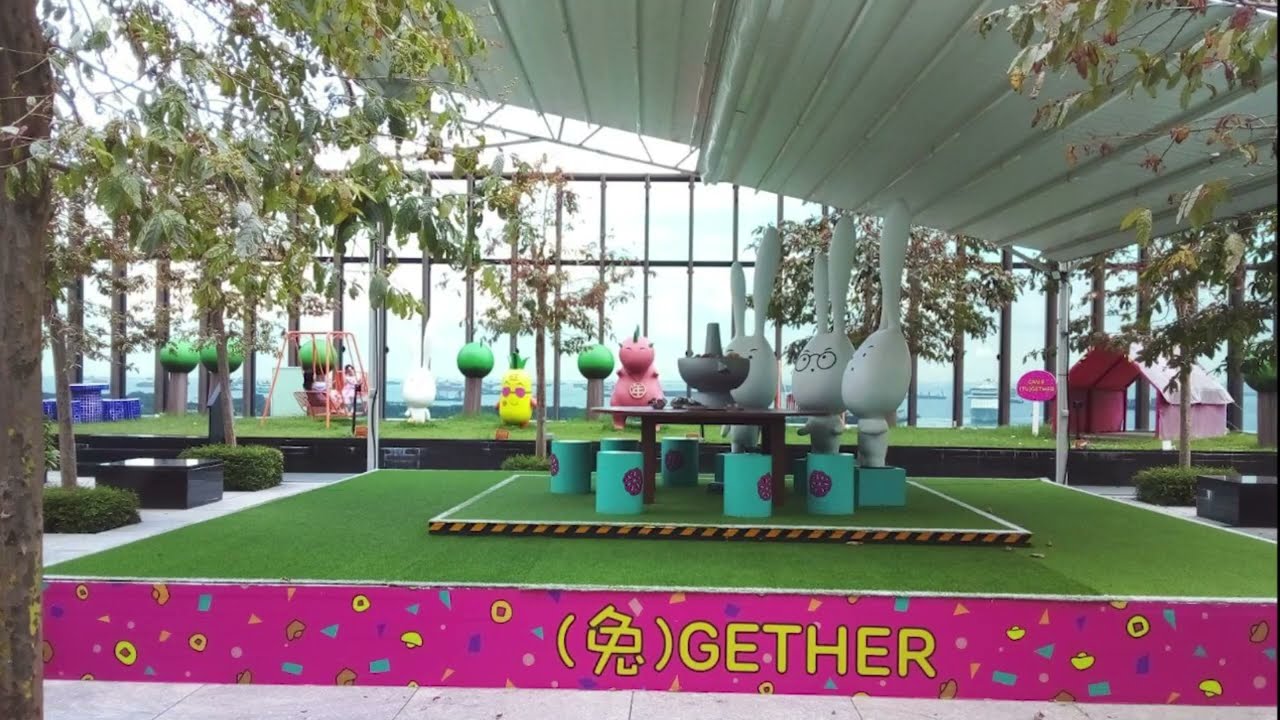The image captures an intricately detailed indoor space that combines elements of a greenhouse, playground, and courtyard. In the foreground, a vivid pink banner with yellow text can be seen, featuring an Asian character within parentheses followed by the word "G-E-T-H-E-R." The banner is adorned with a variety of colorful confetti-like decorations, including blue and peach triangles and squares. 

Central to the scene is a raised platform covered in astroturf, upon which stands an even smaller platform. Atop this, there is a table surrounded by futuristic green chairs. The table is populated with whimsical, cartoon-like sculptures of three white rabbits—one in the middle with glasses—a pink dinosaur or unicorn, and other cartoony figures, possibly including a pineapple. These figures have a playful, almost inflatable appearance, though their material is not clear.

The indoor area is lush with plants and scattered trees, framed by expansive glass walls that feature rectangular metal framing. The slanted roof appears to be made from metal sheets divided by spines and looks as though it may retract. In the background, a swing set adds to the ambience of an indoor park or play area. The setting is filled with natural light, suggesting a bright, airy atmosphere perfect for a whimsical gathering or family-friendly event.